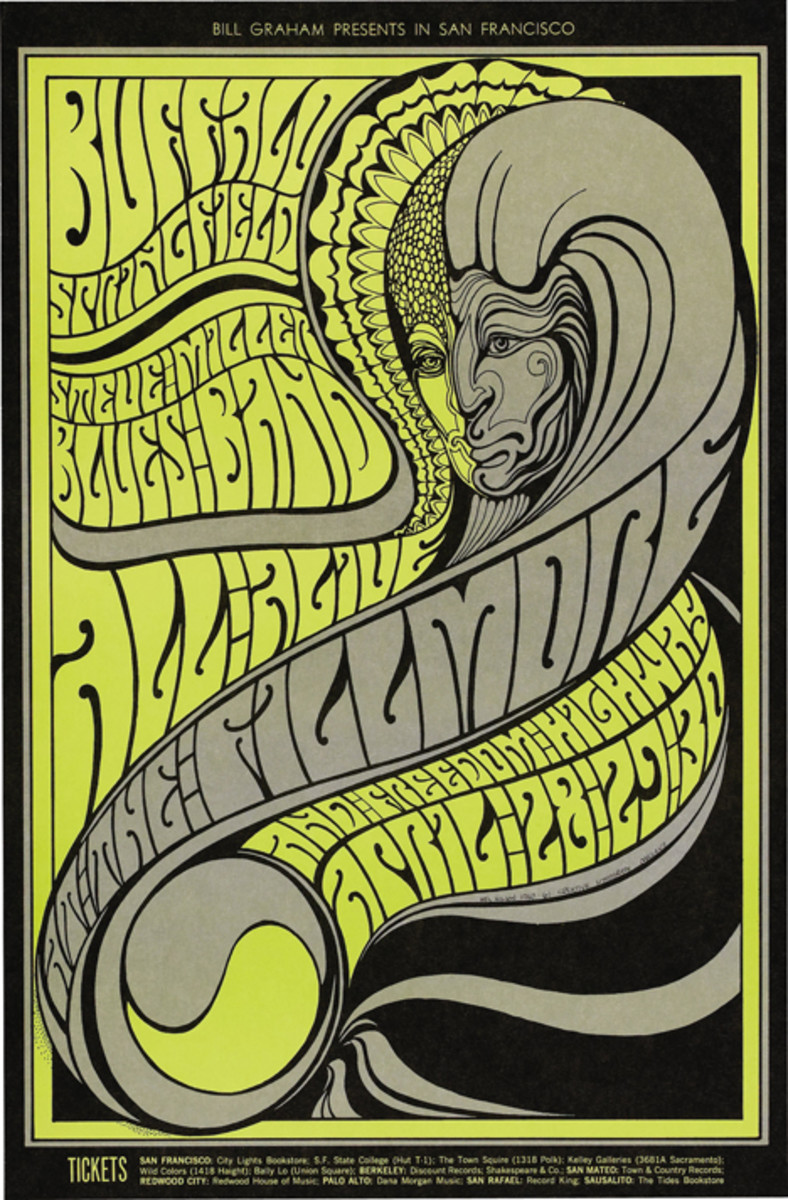This is a detailed description of a promotional poster, possibly for an event or show presented by Bill Graham in San Francisco. The vertically oriented poster features a prominent black background with vivid yellow and gray accents. At the top, in small yellow text, it reads "Bill Graham presents in San Francisco." 

The central image on the poster appears to be an abstract, humanoid face with long, flowing hair that swirls and curves, reminiscent of both ram's horns and scales or feathers, creating a dynamic and curvaceous effect. The face might even suggest a dual perspective, with one part depicted in a side profile.

Encircled by a layered border with sections in gray and yellow, the intricate head design captures attention. At the very bottom, the poster also mentions "tickets" and specifies "San Francisco City Lights Bookstore," alongside additional cities in fine print, such as Redwood City, Berkeley, Palo Alto, San Rafael, San Mateo, and Sausalito. While much of the smaller text is unreadable, the overall aesthetic is a striking combination of abstract artistry and promotional details.